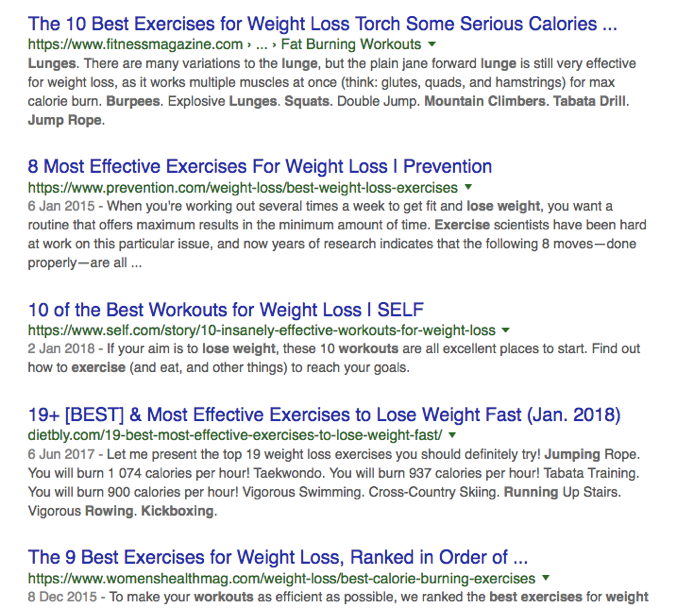The image is a vertically rectangular partial screenshot capturing search result listings, likely from a Google search. The results are displayed on a white background, with each listing presented in a structured format: the title of the website in blue, the URL in green below the title, and a brief description in black text. The captured contents include:

1. "The 10 Best Exercises for Weight Loss" 
2. "Torch Some Serious Calories"
3. "8 Most Effective Exercises for Weight Loss and Prevention"
4. "10 of the Best Workouts for Weight Loss | SELF"
5. "19+ Best and Most Effective Exercises to Lose Weight Fast | January 2018"
6. "The Nine Best Exercises for Weight Loss, Ranked in Order of..." (The complete title is cut off by an ellipsis).

This screenshot specifically captures the list of exercise-related articles, emphasizing their relevance to weight loss strategies. No browser or search engine interface elements are visible, making it unclear which platform the search results are from.